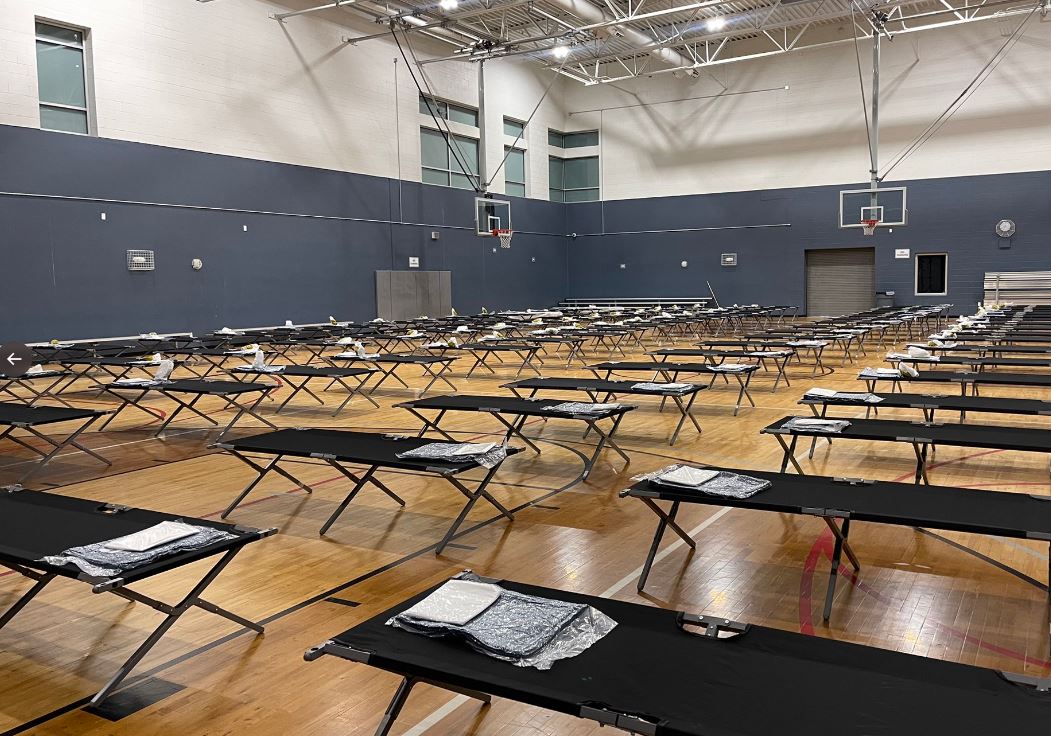This photograph captures a gymnasium repurposed as a temporary shelter. The gym's wooden floor is lined with rows of black foldable camping cots, arranged in at least four or five uniform rows, creating a structured grid. Each cot is topped with an unfolded sheet positioned towards the head, suggesting readiness for immediate use. The scene is devoid of people, emphasizing the stark, utilitarian setup.

The gymnasium walls are painted blue at the bottom and transition to white at the top, creating a clean, institutional feel. Notable features include two basketball hoops mounted on either side of the gym, indicating its primary function as a sports facility. The overall atmosphere suggests a somber setting, likely intended to provide temporary accommodation for people in need.